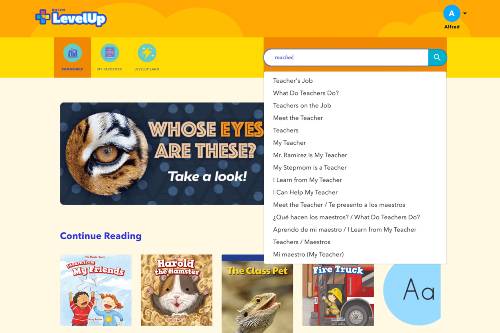The image features a brightly colored design with a predominant orange border at the top. Central to the image is a directional pad resembling those found on video game controllers, depicted in blue, yellow, and purple hues. Bold text over the directional pad reads "Level Up." In the top right corner, there is a notable blue circle containing the letter "A."

Below the "Level Up" text, there are three blue circles, each with different icons in the center. Due to the slight blurriness of these icons and the text underneath them, the specific details are not clear. Adjacent to these elements, a close-up of a tiger's eye is displayed with the text "Whose eyes are these? Take a look."

Additionally, the image contains a search bar situated above a drop-down menu listing several titles such as "Teacher Jobs," "What the Teacher Do," "Teacher on the Job," "Meet the Teacher," and "Teacher My Teacher." Below this menu, the phrase "Continue Reading" is present.

At the bottom of the image, four distinct book covers are displayed, featuring titles such as "Harold the Hamster," "The Class Pet," and "Fire Truck."